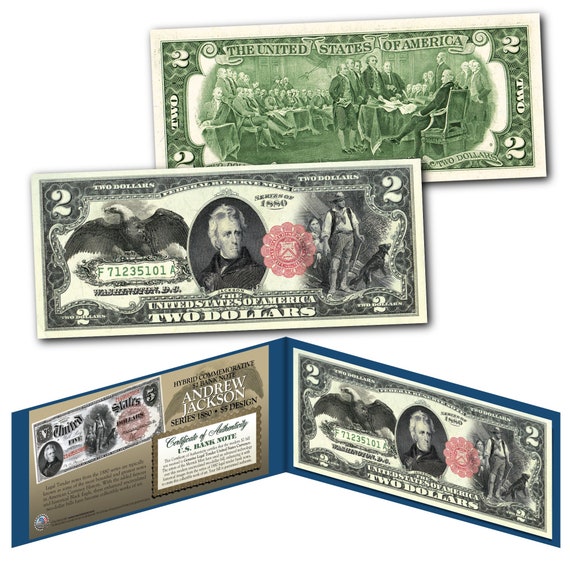This image showcases a collectible $2 bill featuring Andrew Jackson, presented in a blue, protective casing with a certificate of authenticity. The photograph displays both the front and back sides of the bill in detail. On the front, the bill prominently features Andrew Jackson's portrait, the number "2" on both left and right sides, and a red Treasury stamp on the right. The serial number "F71235101" is printed in green beneath a bald eagle illustration. The back side exhibits a detailed scene of the signing of the Declaration of Independence, with the Founding Fathers gathered and George Washington at the center. The bill is mainly white or beige in color, with large green number "2"s on either side and the word "TWO" in white running vertically. The entire setup appears to be a rare, collectible version of the $2 bill, potentially a newer mint edition, encased for preservation.